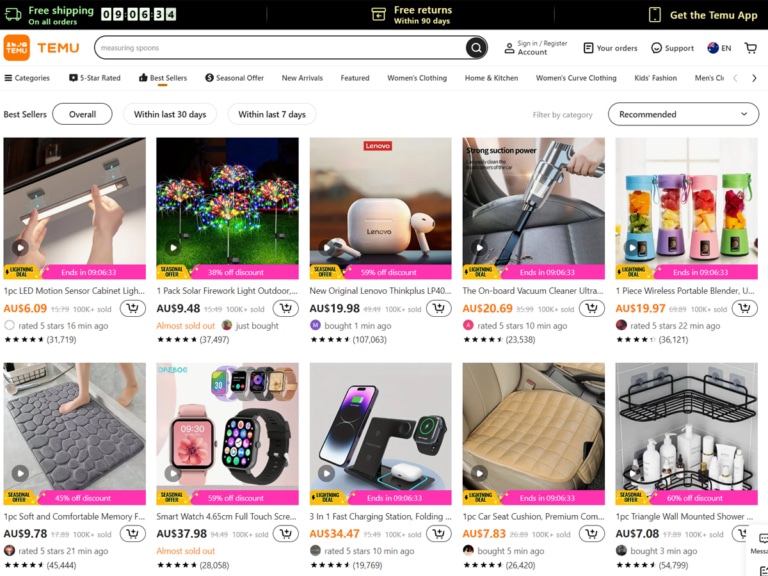This image showcases a promotional banner at the top with a black border that highlights key offers: "Free shipping on all orders" and "Free returns within 90 days." On the right side, there's a call-to-action to "Get the Temu app." Adjacent to this, on the left, is the Temu logo and icon. Below the logo, there's a search box, and to the right of it, a menu with links to "Your Order," "Support," and various product categories, including "Five Star Rating," "Seasonal Offer," "Featured," "Home and Kitchen," and "Women's Clothing."

Beneath this section, there are ten thumbnail images of items for sale, each with a product name and description below it, though the text is too blurry to read clearly. The top-left thumbnail displays a small light fixture being installed, while the image to its right appears to feature outdoor Christmas lights draped over bushes.